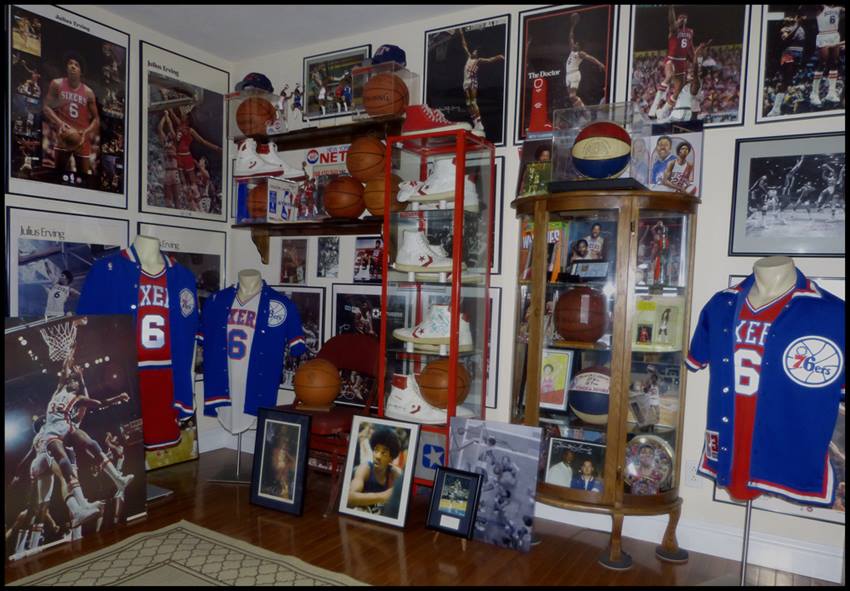This photograph captures an extensive collection of Philadelphia 76ers memorabilia in what appears to be a dedicated room, possibly in someone's home. The room's interior features two white walls and a white ceiling, with a shiny brown wooden floor partially covered by a tan rug. Framed photographs of various basketball players, primarily the Sixers—members of the Philadelphia 76ers—adorn the walls. Among the memorabilia, several photos prominently feature Julius Erving, also known as "Dr. J," depicted in various iconic basketball moments.

The collection is extensive, with several shelves and a curio cabinet displaying numerous basketballs, some of which are signed and encased in glass containers. The display includes three partial mannequins dressed in 76ers jerseys, complete with shorts and matching jackets in red, white, and blue variations. Multiple pairs of sneakers—which may have been worn by players—are also visible on shelves and in a tall, narrow case.

The room exudes a sense of nostalgia and admiration for the sport, with additional memorabilia such as posters, team uniforms, and jackets contributing to the theme. The meticulous arrangement of items and the variety of memorabilia suggest that this is a cherished collection, likely assembled by an avid 76ers fan.